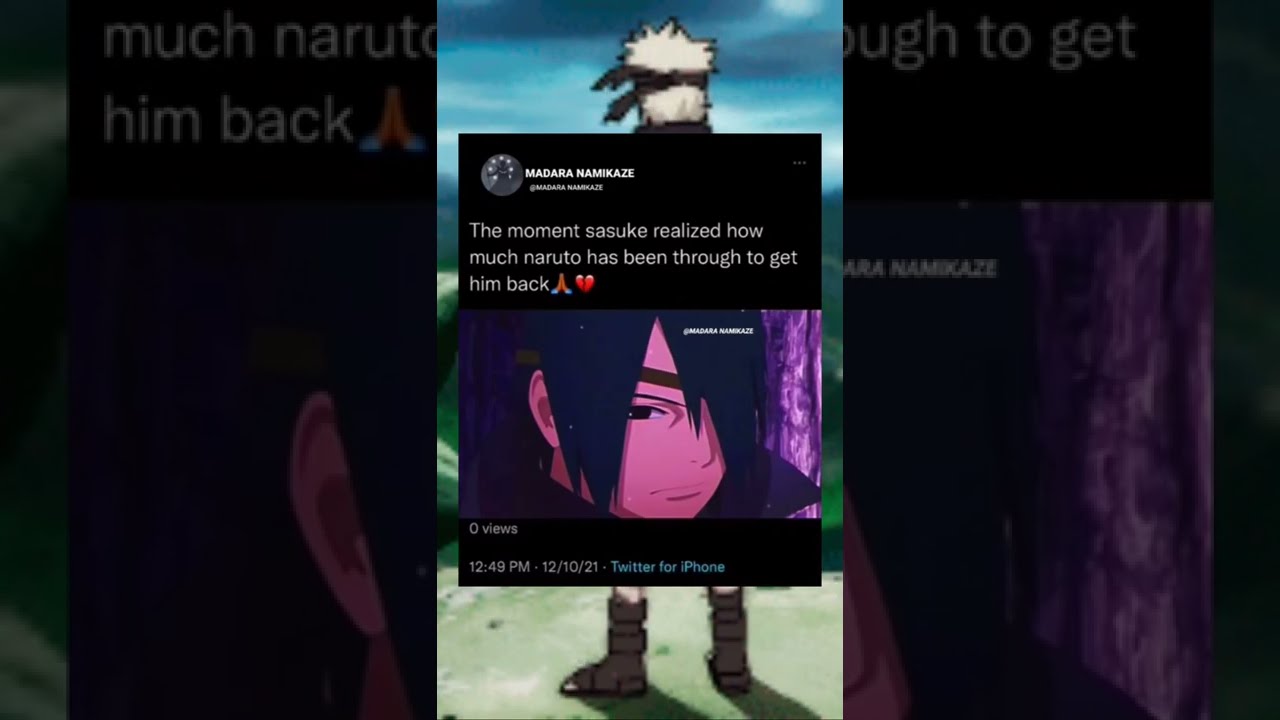The image appears to be from a video game or animated series featuring characters from Naruto. It depicts a man with white hair and a headband standing on what looks like a mountain, seen from the back with a bandana blowing in the wind. Overlaid on this scene is a social media post by "Madara Namikaze," timestamped at 12:49 PM on December 10, 2021, from Twitter for iPhone with zero views. The post contains a three-panel meme format: the central panel shows a close-up of Sasuke with a serious expression and the caption, "The moment Sasuke realized how much Naruto has been through to get him back," accompanied by prayer and broken heart emojis. The side panels are zoomed-in, less clear repeats of the central image, framing the meme. The background behind the post is bright purple, and the character in the foreground is wearing brown hiking boots.